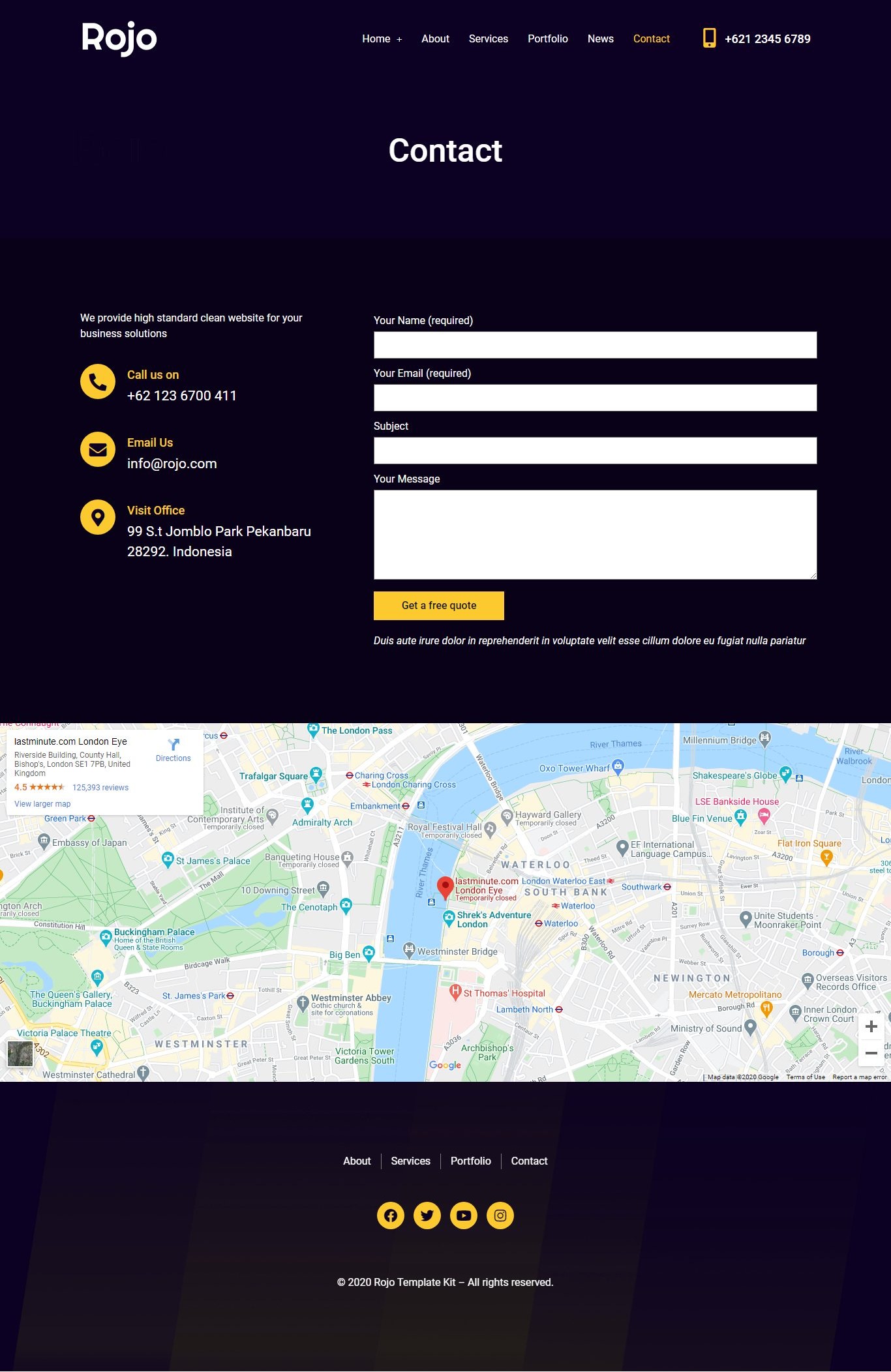This is a detailed screenshot of a webpage named "Rojo," displayed on a black background. The screen is divided into three distinct components:

1. **Contact Section**: The upper portion of the screen features a contact form set against a black background. The contact form contains four white input fields for users to provide their name, email address, subject, and message. There is a yellow pill-shaped button below the message field for submitting the form.

    - On the left side of this section, there are several contact details:
      - A telephone icon with a corresponding phone number.
      - An email icon, represented by a yellow circle with a black envelope, followed by an email address.
      - A location marker icon, under which there is a clickable map.

2. **Map Section**: The middle portion of the screenshot displays a map depicting a city split by a river. The right bank of the river has a red marker indicating the office's location. 

3. **Social Media and Navigation Section**: The lower portion of the screen features a broad band with social media links, represented by familiar icons such as "F" for Facebook and "bird" for Twitter. Below these icons, there are navigation links to "Services," "Portfolio," and "Contact" sections for easy access.